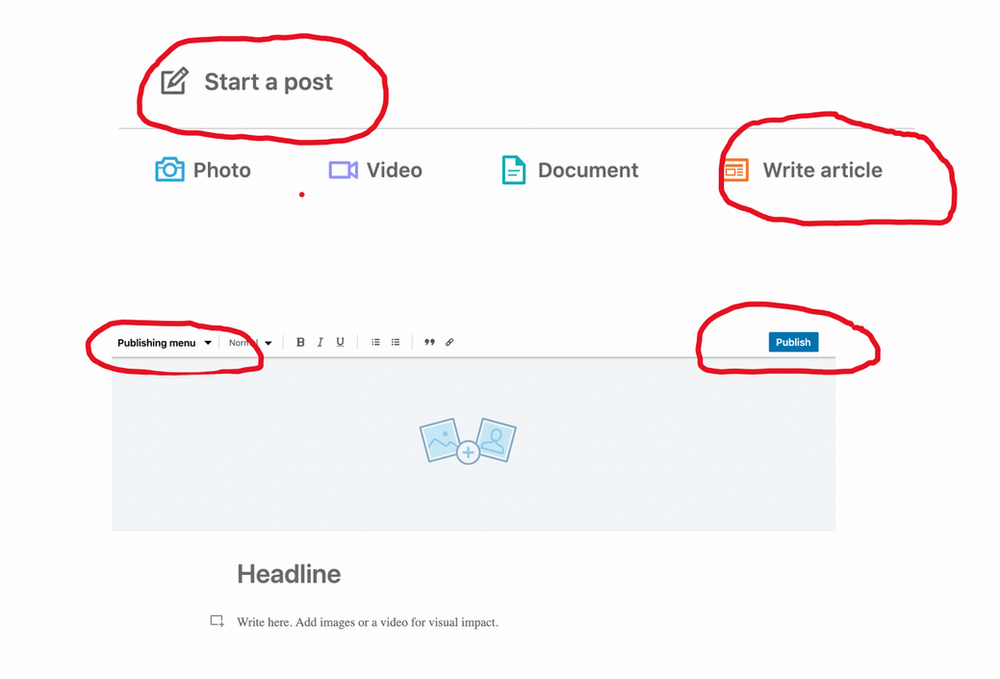The image showcases a webpage interface with various interactive elements for creating and publishing content. 

At the top, there is a prominent white square featuring another smaller white square inside it. Within this smaller square, the text “Start a post” is clearly visible. The icon of a piece of paper with a pen accompanies the text, and both are encircled in red marker, drawing attention to this area.

Below this section, there is a gray horizontal line. Underneath the line, it reads “Photo video document or write article,” with “Write article” also circled in red marker, emphasizing this option.

Further down, the text “Publishing menu” is displayed. This section contains two blue boxes set against a gray background. These boxes appear slightly slanted and not perfectly straight. Between them, there is a plus sign inside a white circle. 

On the right side of this section, the word “Publish” is displayed in a blue rectangular box with white letters, which is also circled in red marker. Beneath this, a text field labeled “Headline” is present. Additionally, there is a note within a box stating, “Write here in images or a video for visual impact.”

This detailed layout captures the essential elements of the webpage, guiding users through the process of starting a post, adding content, and eventually publishing it.